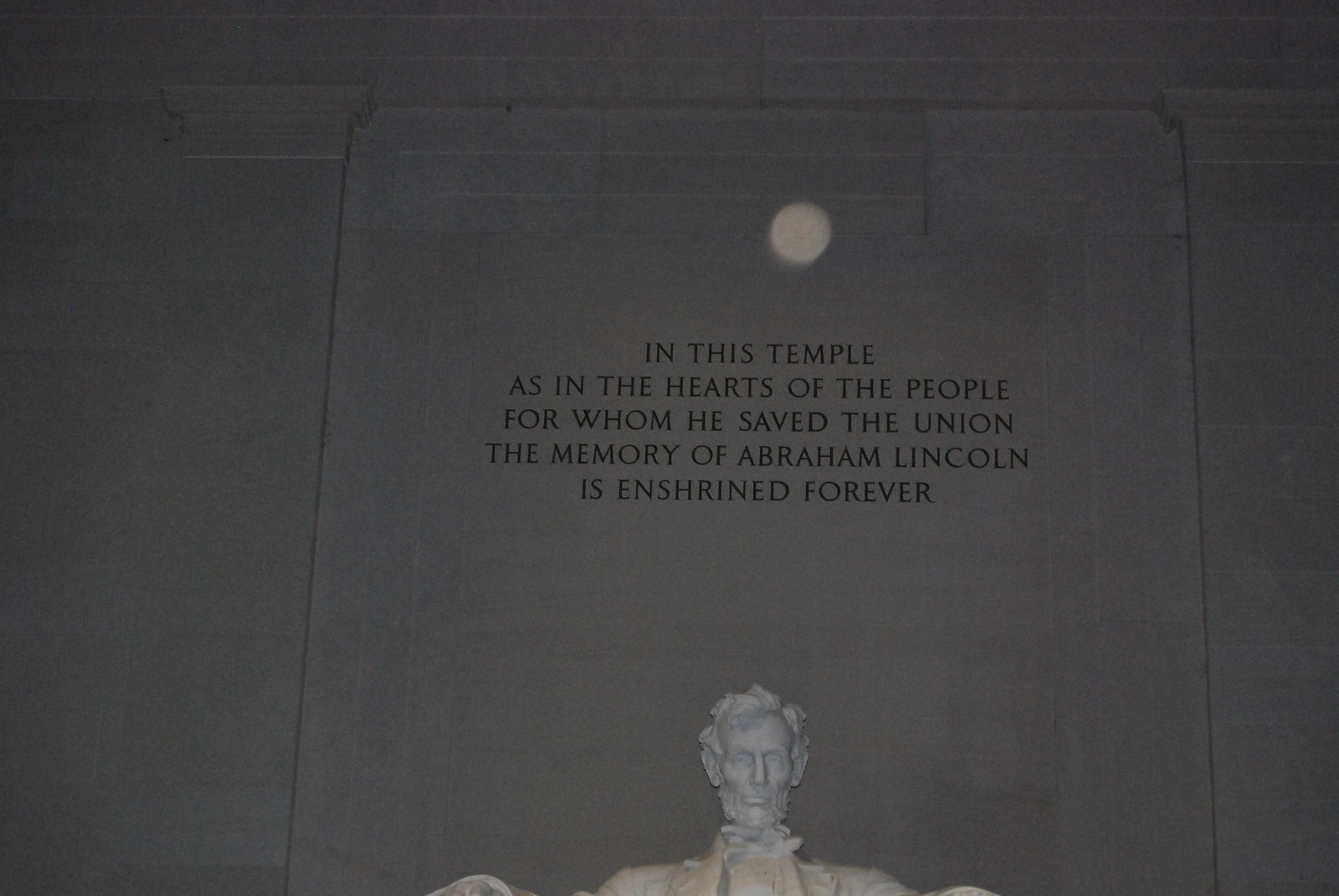This detailed photograph captures the iconic statue of Abraham Lincoln seated in a distinguished pose at the Lincoln Memorial in Washington, D.C. The statue, made of white marble, shows Lincoln seated in a large armchair, hands resting on the chair's arms, and gazing straight ahead with a composed expression. His hair appears somewhat tousled, and he is depicted without a hat, dressed in a bow tie, a tuxedo jacket, and a tuxedo shirt. He has a solemn face, with no smile and facial hair framing his resolute demeanor. 

The image prominently features the engraved inscription above the statue, which reads, "In this temple as in the hearts of the people for whom he saved the Union, the memory of Abraham Lincoln is enshrined forever." This inscription reflects the monumental reverence for Lincoln, celebrating his enduring legacy in the hearts of the nation. The upper part of the statue, particularly Lincoln's head and chest, are clearly visible in the lower portion of the photograph, which is characterized by a gray and dark tone. Just above the inscription, there is what appears to be a reflection, possibly of the moon, adding a serene and contemplative dimension to the image. The Lincoln Memorial, contrary to some beliefs, serves solely as a monument and not as Lincoln's final resting place.